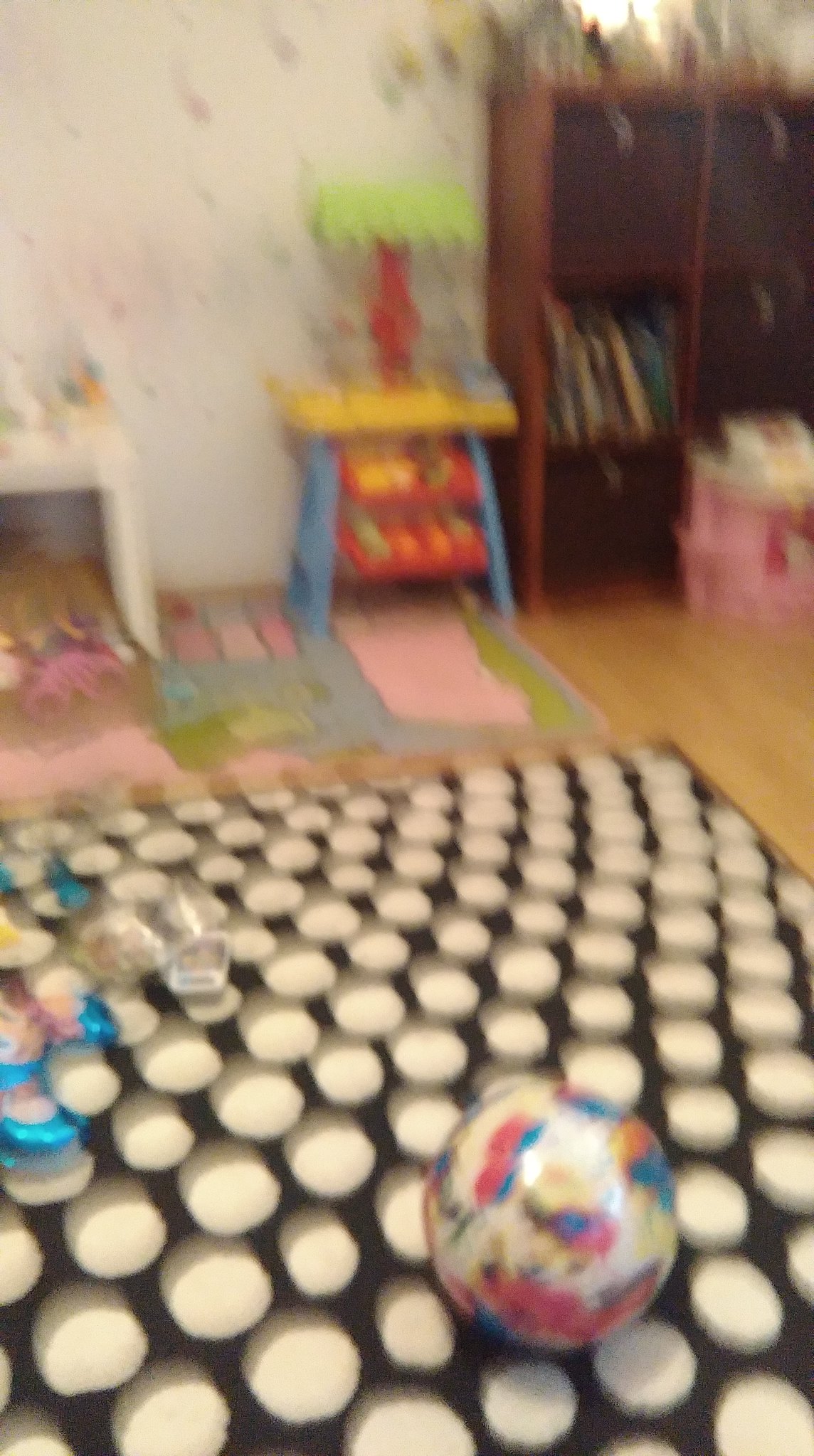This image, though significantly out of focus, depicts an indoor children's play area. The foreground prominently features a large black play mat adorned with white circular polka dots. Scattered on the mat are various toys, the most noticeable being a substantial, plasticky ball detailed with pink and blue trim on a white background, roughly the size of a basketball. Though the image blurs some of the smaller toys, their presence adds to the playful clutter.

Extending into the background, the laminated wooden floor leads to a white wall, which is decorated with numerous stickers. A brown bookcase sits against the wall, stocked with children's books and additional toys. Further into the room, a toy structure resembling a tree and a pink dollhouse can be discerned among other playthings. A variety of colored items—green, pink, blue—dot the room, adding to the vibrant and lively atmosphere. A plastic white table, typically used by small children for activities like eating or drawing, is also visible within this engaging and playful space.